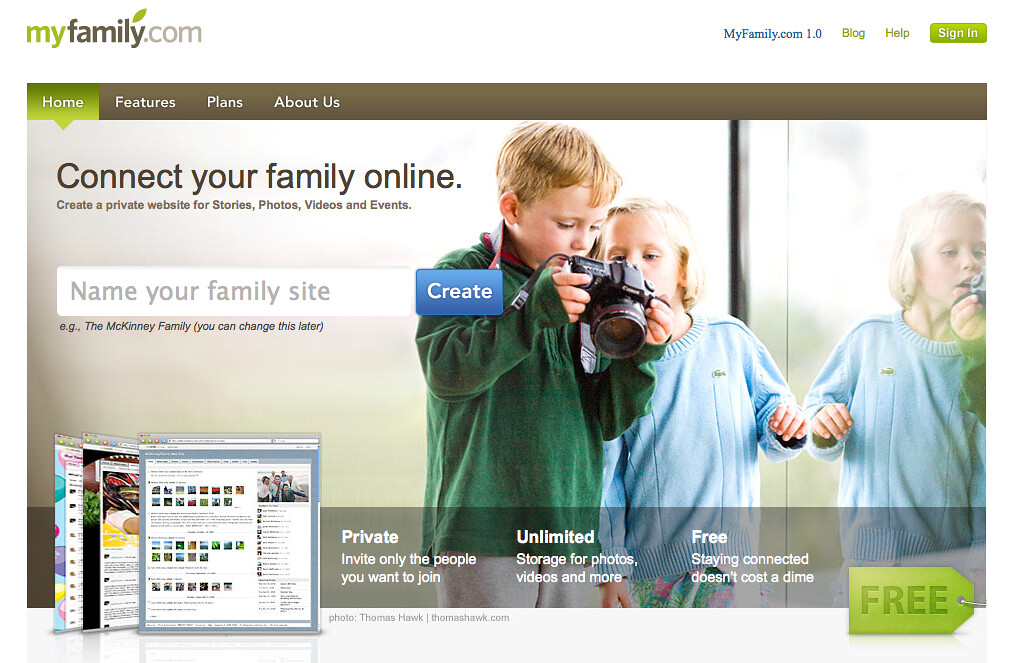This image is a detailed screenshot of the homepage of MyFamily.com, a website designed to connect families online. The website's name and logo "MyFamily.com" are prominently displayed in various shades of green and gray in the top left corner, with "MyFamily.com 1.0" listed in the top right. The header menu includes options for "Home," "Features," "Plans," and "About Us," with "Home" currently selected in a green rectangle.

The main content of the page features a headline that reads, "Connect your family online." Below this, the subheading encourages users to "Create a private website for stories, photos, videos, and events." In the center, there is a text box prompting users to "Name your family's site," accompanied by a "Create" button.

Overlaid on this central content is a background photograph of two young children, a boy and a girl, both fair-skinned. The boy, who has blonde hair and is dressed in a green hoodie and white trousers, is holding a Canon DSLR camera. A girl, slightly shorter, with light reddish hair, stands next to him in a blue sweater and colorful pants. Both children are intently looking at the camera's screen. Their reflections are partially visible in what appears to be a window or mirror to their right.

At the page's bottom, key features of the service are highlighted: "Private" - inviting only those you want, "Unlimited" - offering boundless storage for photos and videos, and "Free" - emphasizing that staying connected comes at no cost. Additionally, there are examples of family site designs depicted as small images of computer screens on the left side of the page. Lastly, a footer note credits the photo to Thomas Hawk, with a small tag reading "feet" in the bottom right corner.